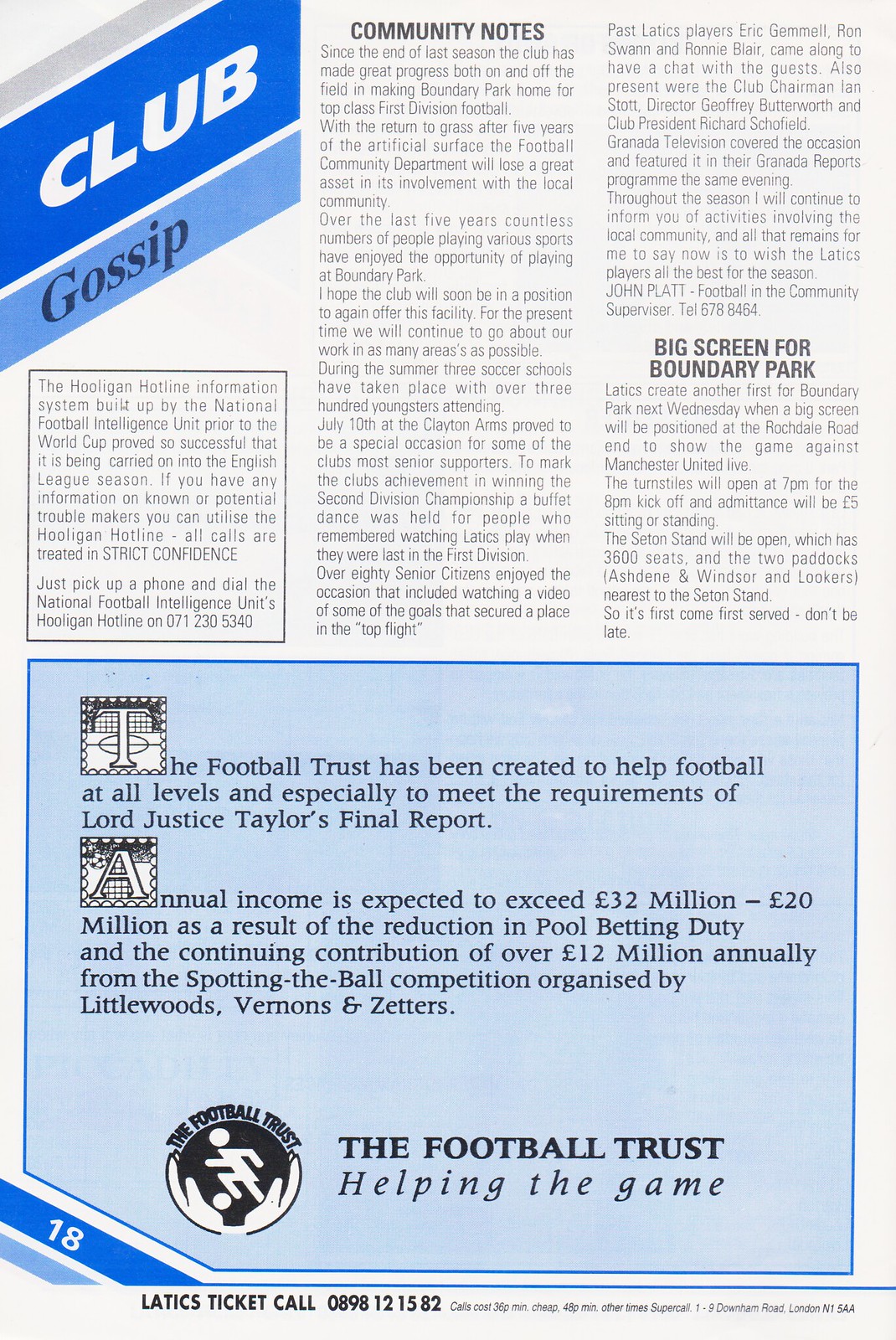In the image, we see a page from what appears to be a newspaper or magazine prominently displaying text sections. At the top, there is a heading titled "Club Gossip," followed by "Community Notes." Below these sections, there's an article titled "Big Screen for Boundary Park." Further down, another heading reads, "The Football Trust has been created to help football at all levels and especially to meet the requirements of Lord Justice Taylor's final report.” The text mentions that the annual income from the Football Trust is expected to exceed £32 million, with £20 million resulting from the reduction in pool betting duty and over £12 million annually contributed through the Spotting the Ball competition, organized by Littlewoods, Vernon's, and Zetter’s. At the very bottom, there's a statement, "The Football Trust: Helping the Game," accompanied by the organization’s logo. The page is tinged with hues of tan, gray, blue, off-white, and black, and the entire sheet takes up most of the image, making the detailed print difficult to read.